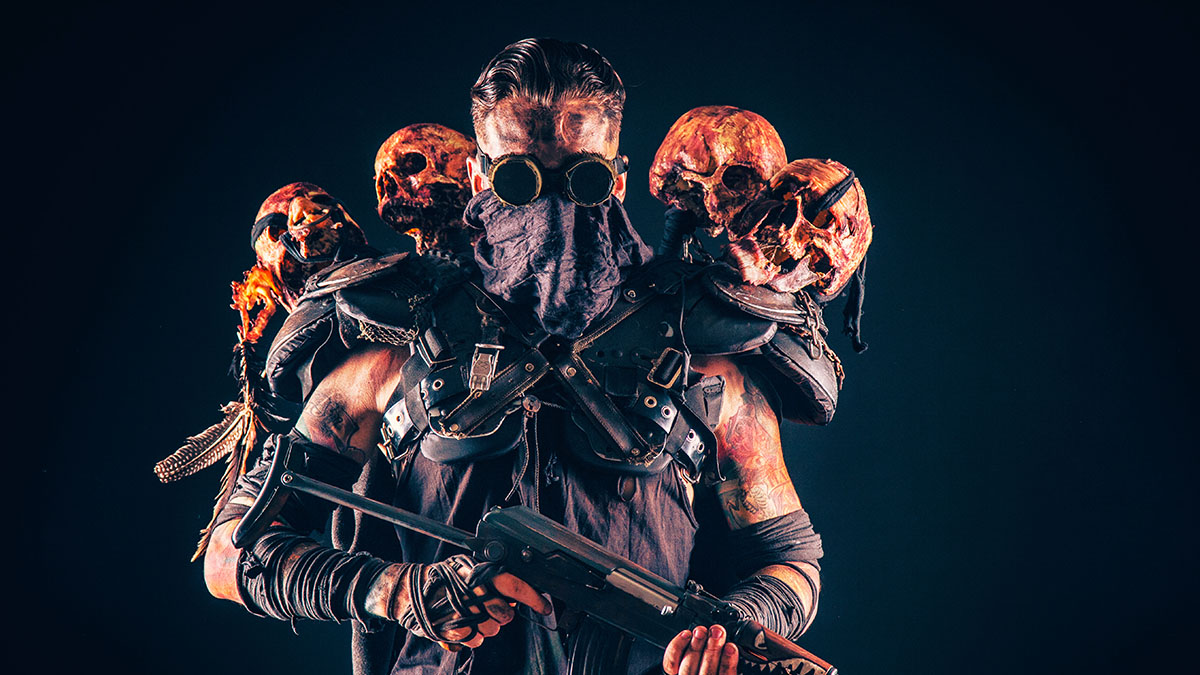This horizontal rectangular image is eerily frightening, with a dark, almost pitch-black background. In the left center stands a menacing figure, clad in post-apocalyptic, marauder-like attire that resembles the character from a dystopian comic book or graphic novel. The man, whose meticulously combed dark black hair contrasts with his rugged appearance, sports welder-style goggles with black lenses and striking yellow rims. His face is partially obscured by a blue mask and a scarf, adding to the aura of mystery and danger.

A mix of leather and fabric adorns his body, with ornamental, post-apocalyptic warrior clothing over his nose, mouth, and shoulders. He grips a black automatic weapon with gloved hands, exuding a sense of readiness for battle. The man's shoulders are particularly striking, each adorned with a pair of bloody, reddish human skulls—two on the right and two on the left—giving a macabre impression that he wears the remains of his victims. The suggestion of fresh blood stains on his gloves and arms further intensifies the gruesome and ominous feeling of this striking image.